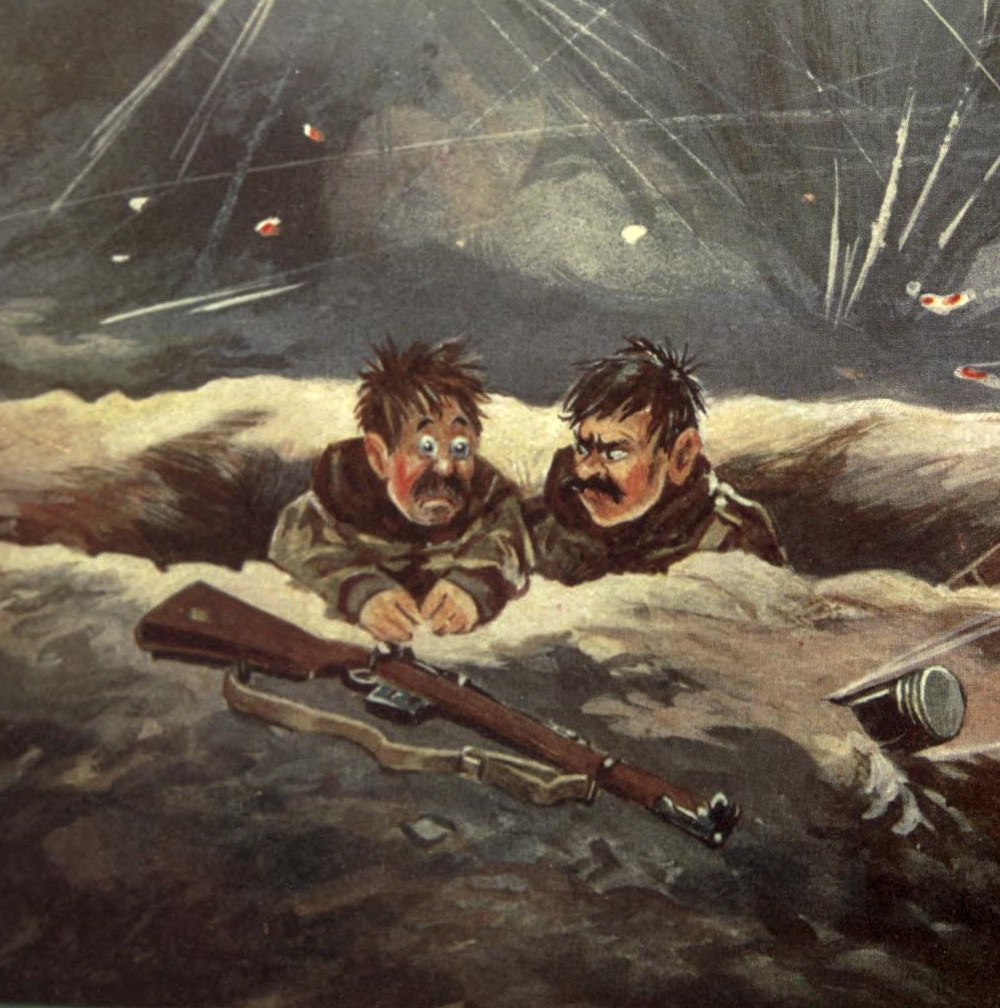This color illustration, rendered in a comic book style, captures a tense scene of two soldiers hunkered down in a foxhole. The square-format image reveals the men from mid-chest upwards, emphasizing their anxious and intense expressions. Both soldiers, marked with grubby faces and unruly hair, sport fur-lined coats and mustaches—one with short brown hair and the other with black hair.

In the foxhole's dirt, a brown rifle with a beige strap lies near a flashlight, symbolizing the readiness and peril of their situation. The soldier on the left has wide eyes and raised eyebrows, glancing anxiously at a freshly landed bomb embedded in the dirt beside the trench. This soldier’s look of alarm contrasts sharply with the soldier on the right's angry scowl directed at his comrade.

Behind them, the sky is dark and filled with smoky haze, punctuated by flying debris and white streaks suggestive of ongoing explosions. The grim setting and the soldiers' tattered appearance hint at the harsh conditions of battle, providing a vivid portrayal of wartime stress and tension.